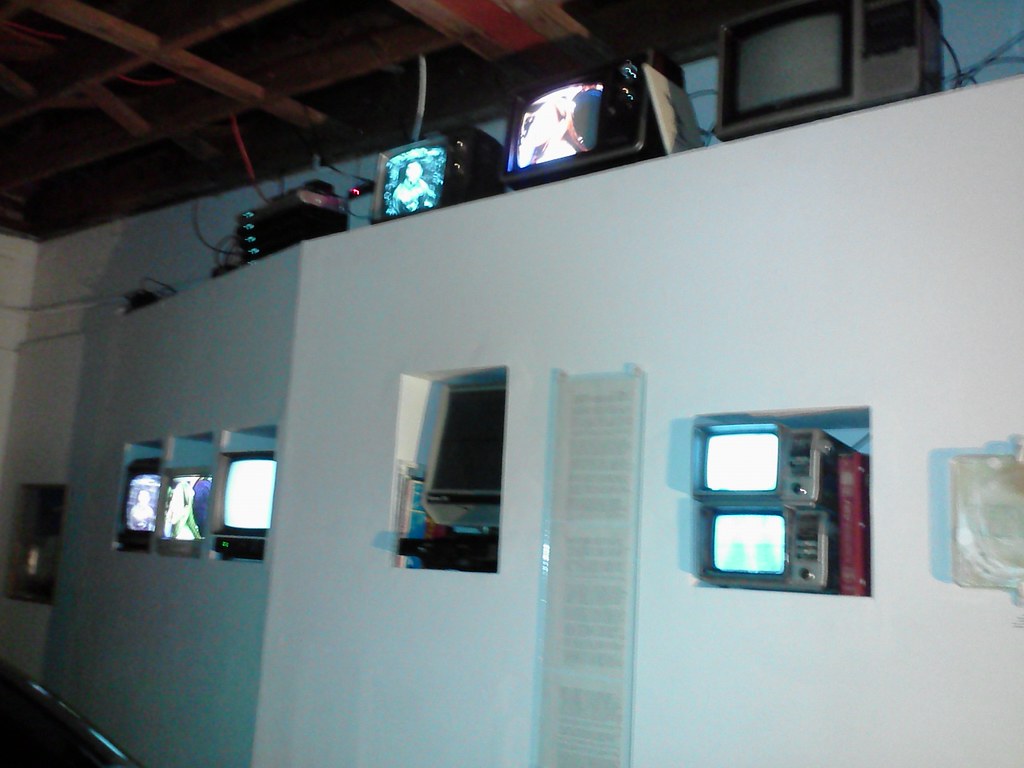The photograph captures a unique wall in a well-lit room with an exposed, beamed wooden ceiling. The white wall has an irregular shape and features multiple recessed niches or cutouts, each housing old-style tube TVs. On the left side, there are three niches, all containing TVs, two of which are displaying programming, while the third shows a white screen. In the middle section of the wall, a cutout holds two mini TVs stacked on top of each other next to a book. Directly above this, a plaque with unreadable text is mounted. There are also additional TVs placed on top of the wall, with two turned on and one off, though the images on the screens are obscured by direct light. A large router with green glowing lights can be seen in one corner. The overall setup suggests a display or exhibit, potentially in a museum, dedicated to vintage televisions.